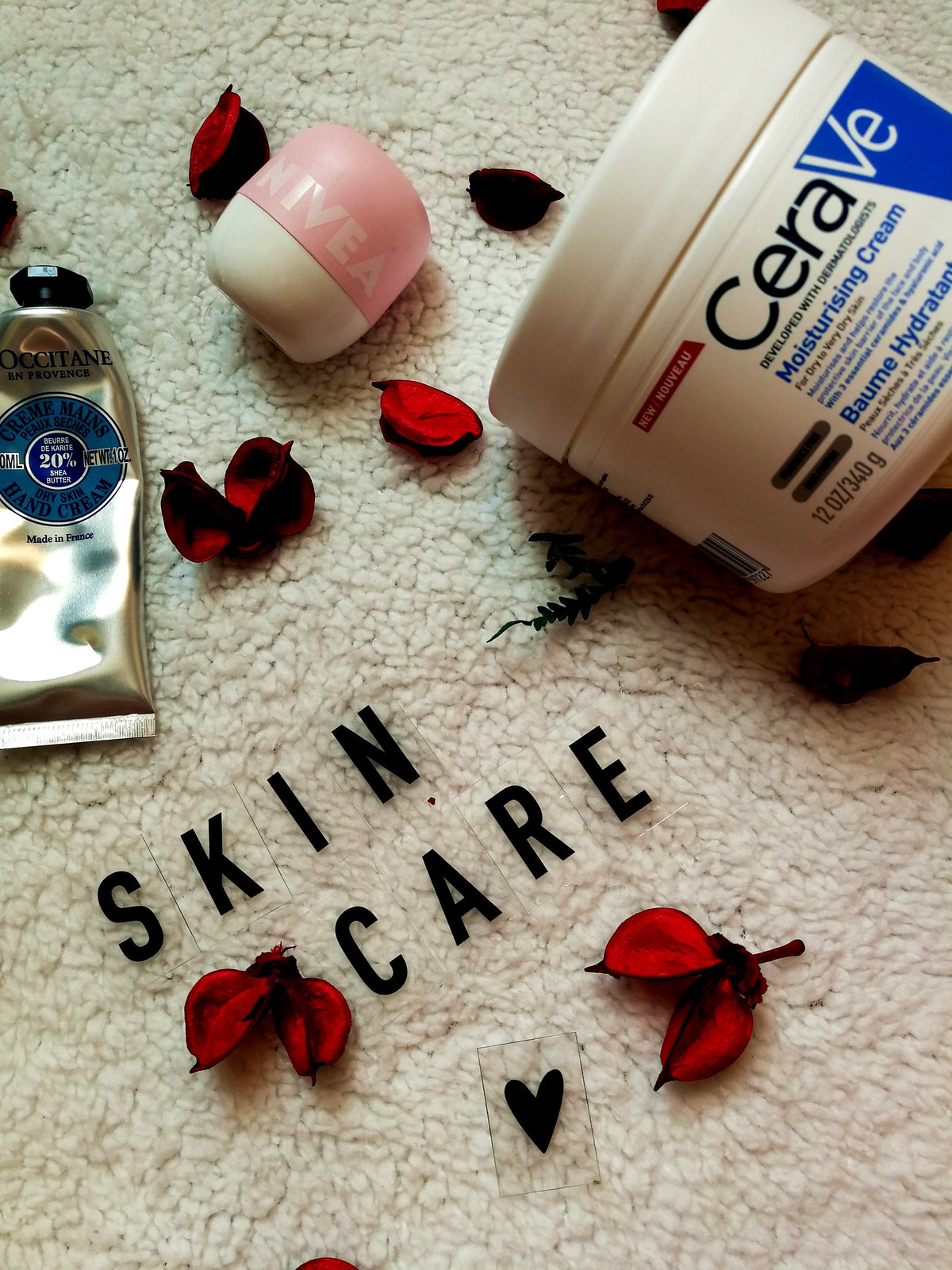In this meticulously arranged photograph, a collection of various skincare products is artfully displayed atop a plush, white, wool-textured carpet, adding a touch of elegance and softness to the background. Scattered throughout the scene are vibrant red flower petals, which provide a striking contrast against the white carpet and enhance the visual appeal.

At the center of the image, clear glass squares arrange to spell out "SKINCARE," accompanied by a black heart symbol beneath, emphasizing the theme of the display. Above this center arrangement, a distinctive container rests, featuring a tan base and a pink top with lighter pink lettering that spells out "NIVEA."

To the left, a sleek, silver tube, reminiscent of a toothpaste tube but actually containing hand cream, proudly displays the label "L'OCCITANE en Provence." This hand cream, noted for its 20% shea butter content, is described as being specifically formulated for dry skin and is marked with a net weight of 0.1 ounces. It is labeled as made in France, signifying quality craftsmanship.

In the upper right corner of the image, a round, white container features prominently with bold lettering declaring it as "CERAVE." The label details that the product is a moisturizing cream developed with dermatologists, tailored for dry to very dry skin. The container holds 12 ounces or 340 grams of this nourishing cream.

Together, these elements create a harmonious and visually pleasing arrangement that underscores the theme of skincare and self-care.